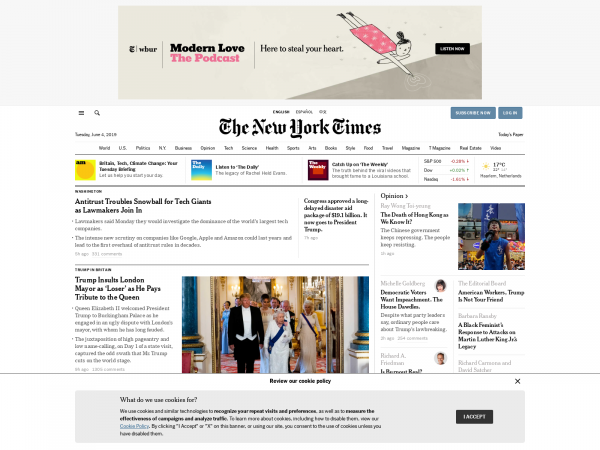The image depicts a news page displayed on an app or web browser screen. At the top, there's a lightly shaded rectangular background. Moving towards the center, there's another shaded area containing small, hard-to-read text. Prominently, it features the title "Modern Love, the podcast" and continues to the right with the phrase "Here to Steal Your Heart." Beneath this title, a drawing of a stick figure-like cartoon woman is noticeable. An angled gray shaded area with a small black section containing text can also be seen. Below this, "The New York Times" is clearly written in the center. Further down, various news articles are displayed, though most headlines are too small to read clearly. Some discernible headlines include "Antitrust Troubles Snowball for Tech Giants as Lawmakers Join In," and "Trump Insults London Mayor at Lesser Event as He Pays Tribute to the Queen," while several other articles remain illegible due to the print size.